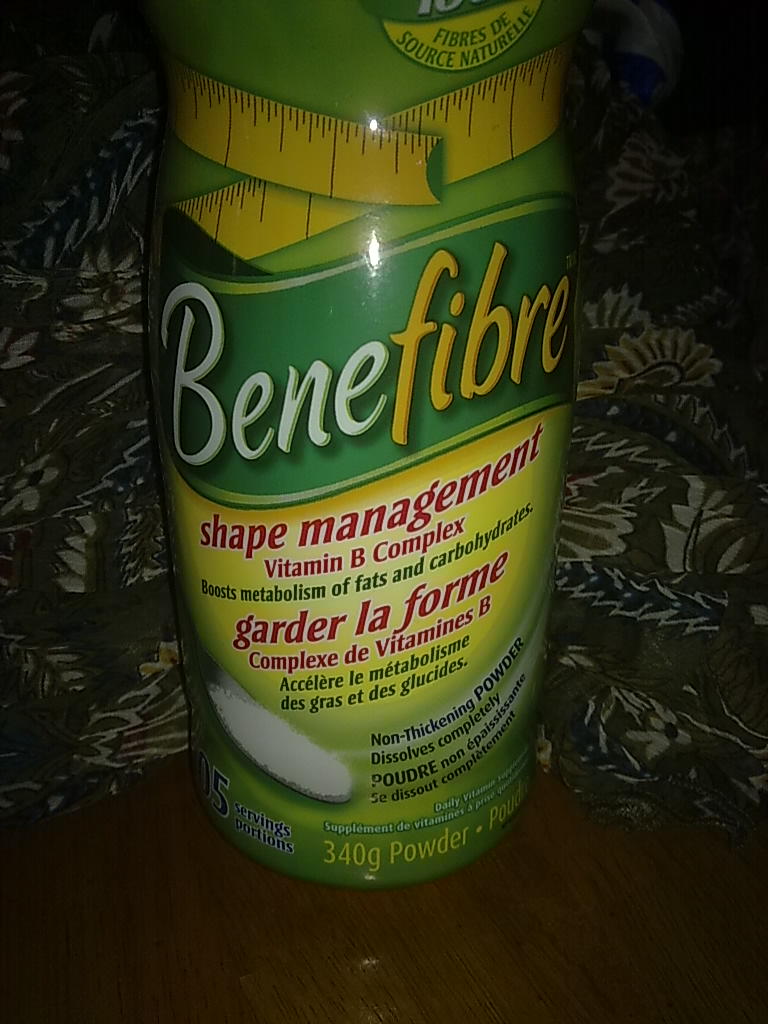The image captures a green, cylindrical plastic container of Benefiber, prominently displayed against a dark background, presumably illuminated by flash as indicated by the slight reflection on the surface. The bottle's color scheme transitions from light green at the top to yellow and back to light green at the base, encircled by a dark green banner in the center. The label reads "Benefibre" in a distinctive blended font: the first part "BENE" is in white while the remaining "FIBRE" is in yellow. Directly beneath, in magenta text, are the words "Shape Management, Vitamin B Complex." Below this, in black text, it reads, "Boost Metabolism of Fats and Carbohydrates." A yellow measuring tape graphic wraps around the upper section, and an illustration of a spoon with the powder is featured at the bottom, emphasizing that it is a non-thickening powder that dissolves completely. Additionally, the label mentions 340 grams of powder and 15 servings on the left-hand side, with the same information repeated in Spanish. The container is positioned on the corner of a dark wooden table, with a background hinting at a blanket adorned with green leaves and white flowers.